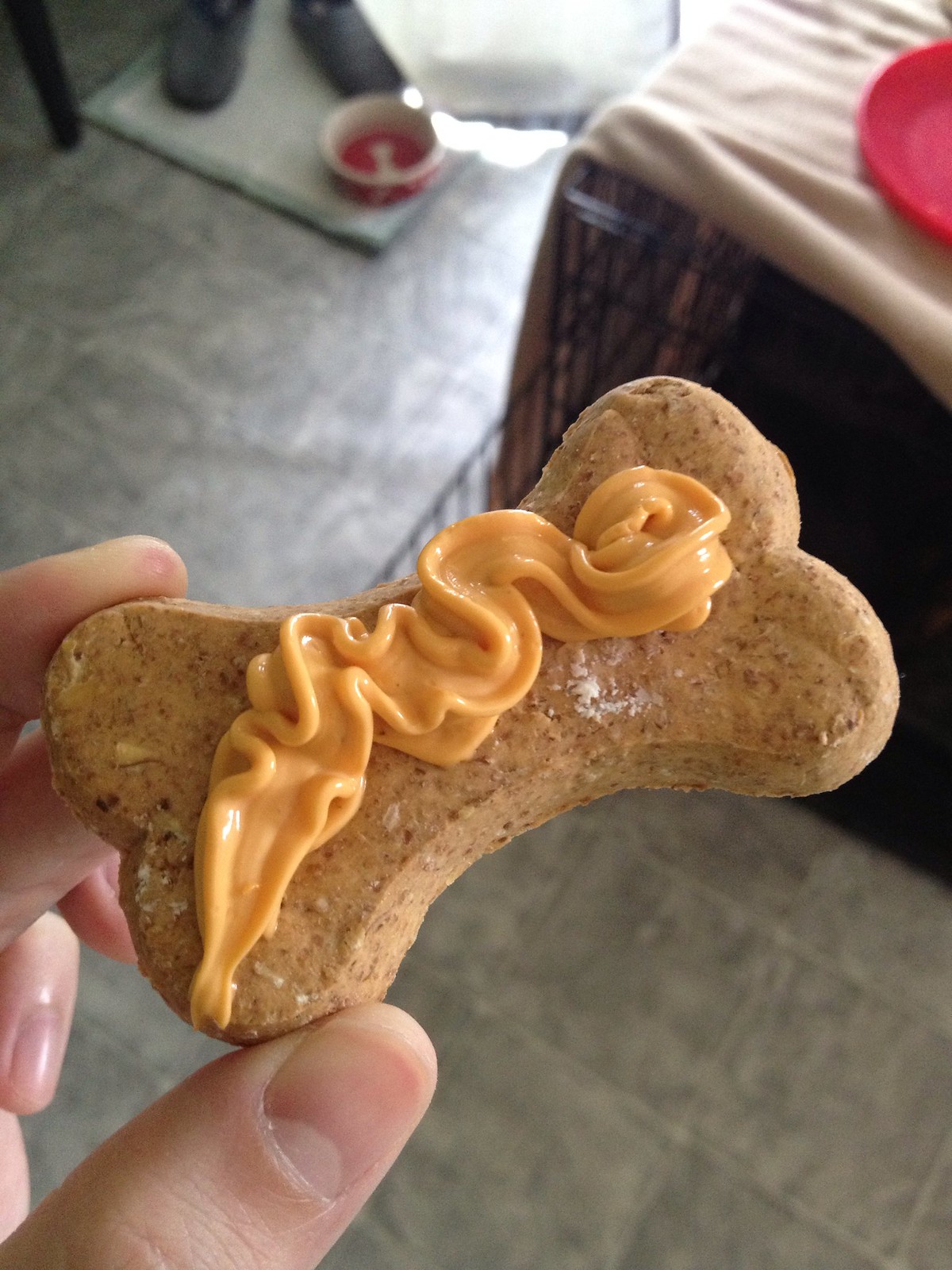The photograph captures a close-up view from above of a light tan dog biscuit shaped like a bone, held at an angle by the left hand of a person with a manicure, suggesting it might be a woman's hand. The biscuit is smeared with a streak of light orange Cheez Whiz and sprinkled with a bit of white powder. The backdrop reveals a gray tiled floor and various dog-related items. To the top right, a black metal dog crate is partially covered by a beige blanket to block sunlight, with a red circular plate resting atop the blanket. The top left corner shows a pair of black shoes or slippers on a gray rectangular mat, next to a red and white dog water bowl.